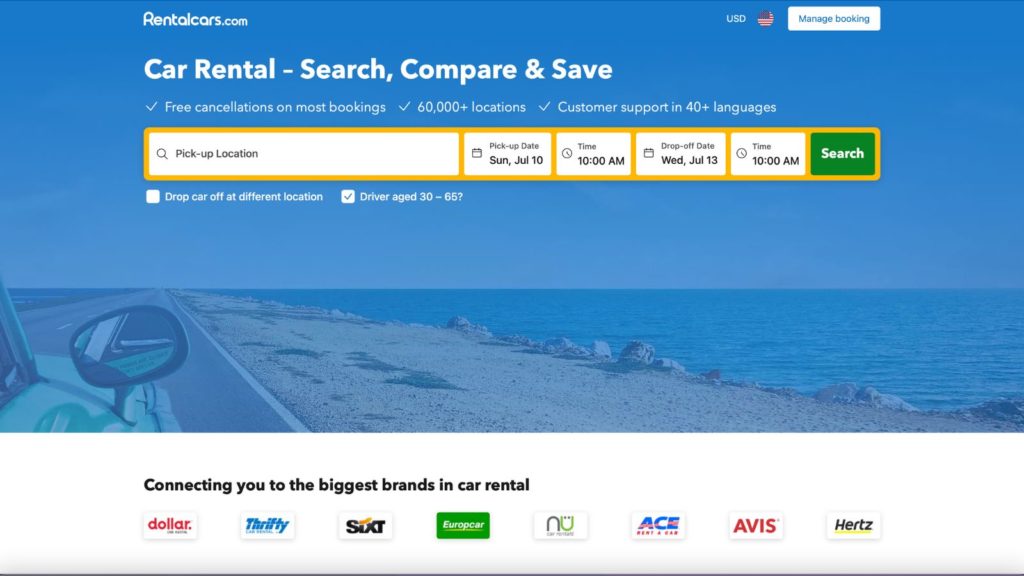A detailed screenshot of the Rentalcars.com website displayed in landscape mode on a laptop screen or computer monitor. The webpage features the Rentalcars.com logo in a custom, distinctive white font positioned near the top left corner of the screen, against a backdrop of a photograph with a blue filter overlay. The photograph showcases the front right corner of a light-colored car, including the side view mirror, situated on an asphalt road that runs parallel to a beach. The landscape moves from gravel and sand to rocks along the shoreline, meeting the ocean or a Great Lake under a blue sky.

The webpage design includes wide vertical margins on both the left and right, with content centered between them. Near the top right, there's an indicator showing "USD" for US dollars with an accompanying American flag icon. Below this, a search box labeled "Manage Booking" is visible.

Prominently displayed in large white letters across the webpage are the words "Car Rental – Search, Compare & Save." Directly beneath, a primary search bar outlined in yellow is split into six sections. Above this bar are features highlighted in white text: "Free cancellation on most bookings," "60,000+ locations," and "Customer support in 40+ languages."

The search bar includes sections for input:
1. "Pick-up location"
2. "Pick-up date," currently set to Sunday, July 10th with a calendar icon
3. "Time" with a clock icon, set to 10 a.m.
4. "Drop-off date," displaying "Wed Jul 13" with a calendar icon
5. "Time," set to 10 a.m.
6. A green search button with white text

Immediately below the search bar are two checkboxes:
- "Drop off car at a different location"
- "Driver aged 30-65?" (checked)

The bottom section of the screen transitions to a white background with black text stating, "Connecting you to the biggest brands in car rental." Below this is a row of thumbnail icons representing eight rental car brands:
1. Dollar (Dollar Rent a Car)
2. Thrifty
3. SIXT
4. Europcar
5. NU
6. ACE
7. Avis
8. Hertz

A thin black line runs across the very bottom of the screen, delineating the end of the page.